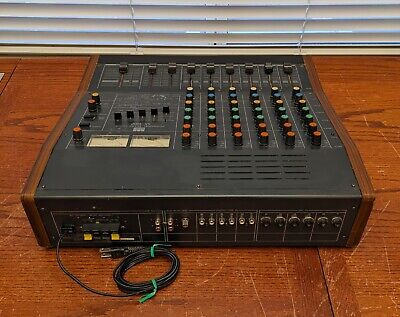This image depicts an electronic device that appears to be an older model switchboard or audio equipment, possibly used in a radio station. The device is situated on a wooden surface and is positioned in front of a window with visible vinyl blinds, allowing bright light to illuminate the scene. The device is flat and rectangular with a black surface bordered by dark wooden edges. On the bottom left, there is a cord, tidily wound and secured with green ties. 

The interface of the device is organized into six rows of colorful buttons, featuring red, green, blue, pink, and white buttons, each with a central hole. Additionally, there are several black knobs arranged diagonally on the left side, and a series of sliders intended for sound adjustments. There are also ports near the bottom for wiring connections. In the center of the device, there are more buttons and switches, all contributing to its complex array of controls.

Overall, the image presents detailed and bustling equipment on a tidy wooden platform, hinting at its utility in audio or video applications.